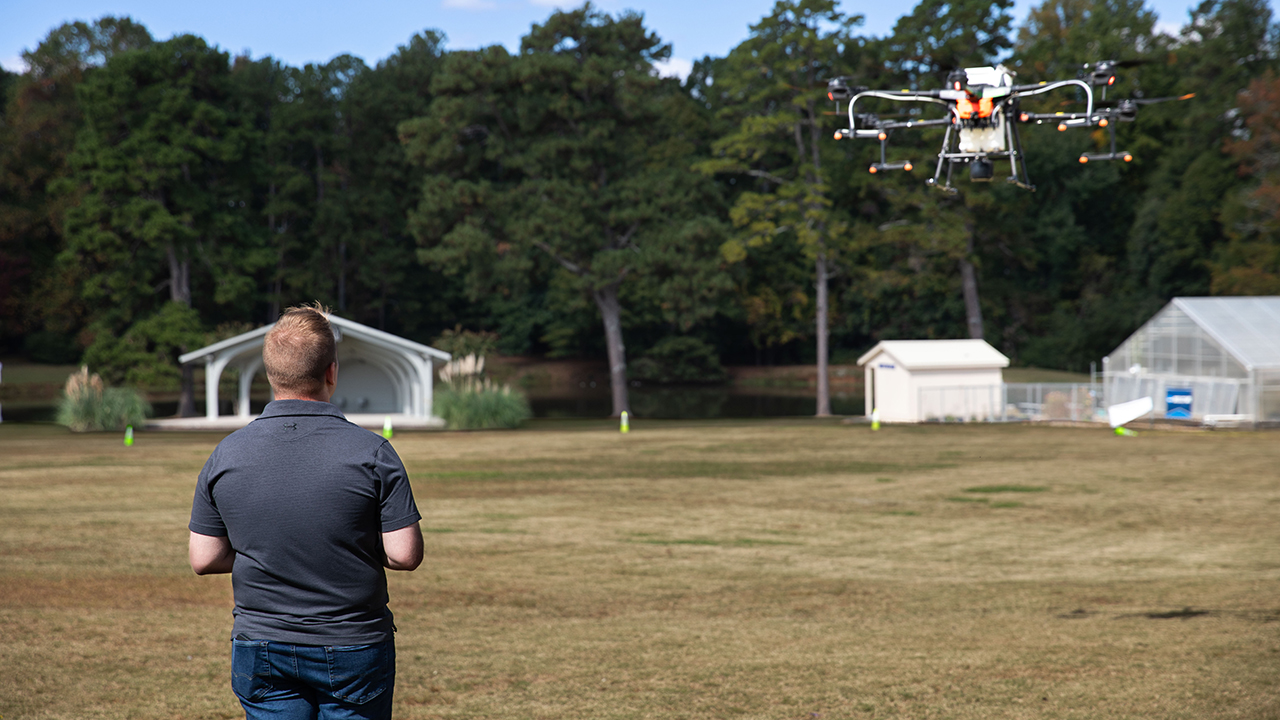The photograph captures a man in a grassy field, piloting a large quadcopter-style drone. The man, sporting a gray polo shirt and blue jeans, has short brown hair and is seen from behind. The field around him is predominantly brown with occasional green spots, and in the background, there's a tree line with thick, dark green foliage. The drone, positioned in the upper right part of the image, is characterized by its substantial size, four propellers, and protectors for landing. It features a white and orange color scheme with a black camera mounted on the bottom. In addition to the natural surroundings, the backdrop includes several structures: a white shed, a gray greenhouse, and a pavilion surrounded by bushes and flowers. The clear blue sky has hints of white clouds. Several neon green cones mark the area, possibly indicating the drone's operational zone.